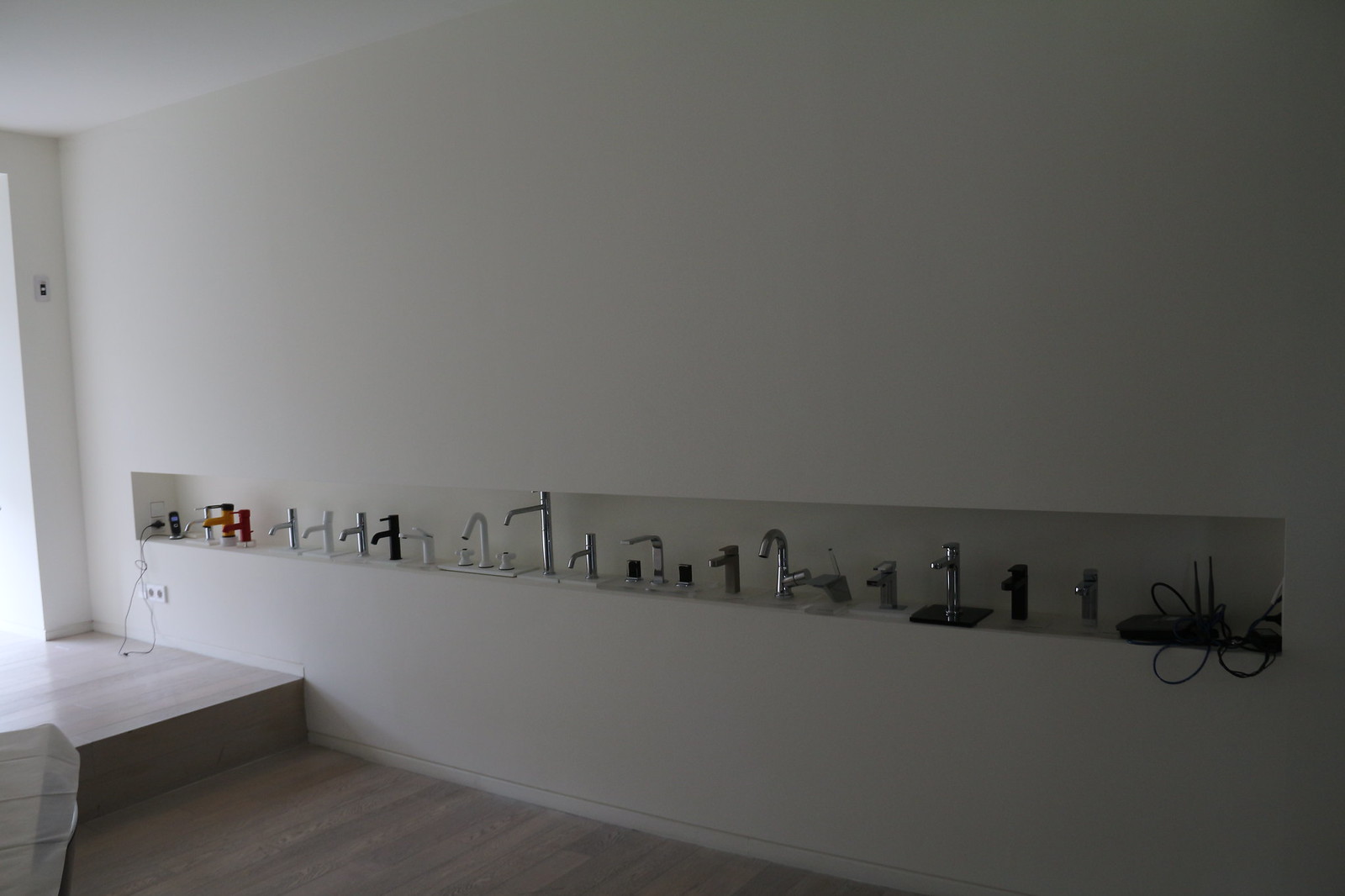This indoor color photograph appears to be taken in a dimly-lit store or museum showcasing a variety of faucets. The subject of the image is a long, built-in shelf recessed into a white wall, which stretches horizontally across the entire space. Inside the shelf, approximately 20 different faucets are meticulously displayed, each mounted vertically. These faucets exhibit a diverse range of designs, colors, and styles, including single stem and dual stem spigots with long and short spouts, in shades of red, black, and metallic finishes.

The room has a wooden or laminate floor, and you can see a slight step down to a lower level, indicating a two-tier layout. Natural light filters in from the left side of the image, possibly through a window or doorway, casting some illumination on the otherwise dark setting. The natural light, although visible, does not reveal the source, and the right side of the image remains quite dark. The overall focus of the photograph is sharp, clearly highlighting the sleek new faucets against the stark white wall. There is no text or wording present in the image.